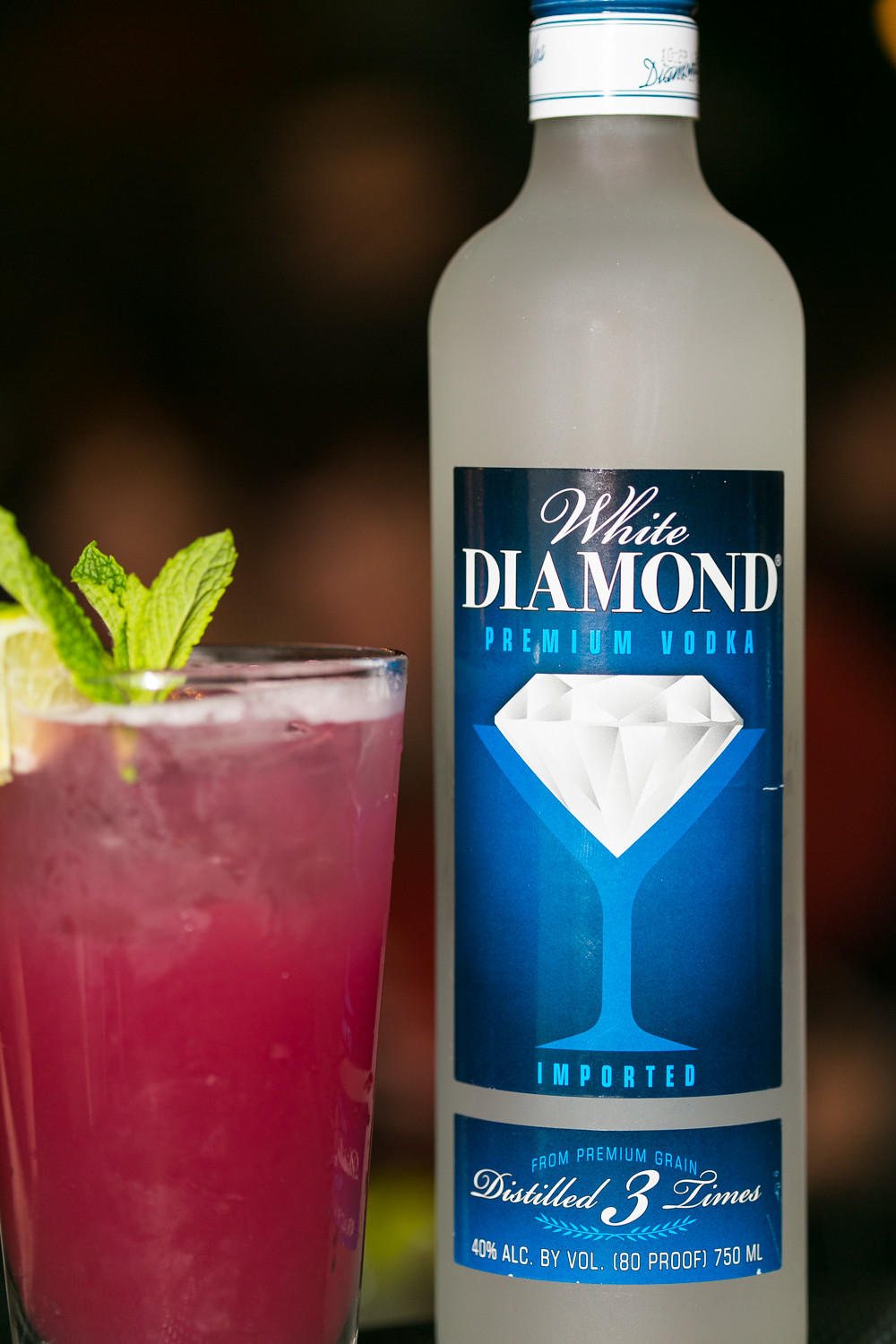The image is a professional advertisement featuring a meticulously arranged display of an adult beverage and a premium vodka bottle against a dark background with indistinct people or brown spots. Dominating the right side of the image is a frosted glass vodka bottle, labeled "White Diamond Premium Vodka" in prominent white letters against a blue backdrop. The label also showcases a large white diamond inside a martini glass and details such as "imported," "from premium grain," "distilled three times," "40% alcohol by volume," "80 proof," and the bottle's capacity of "750 milliliters." Extending from the bottom to the middle on the left side, a chilled clear glass contains a reddish-pink mixed drink with ice, garnished with mint sprigs and a slice of lemon on the rim.